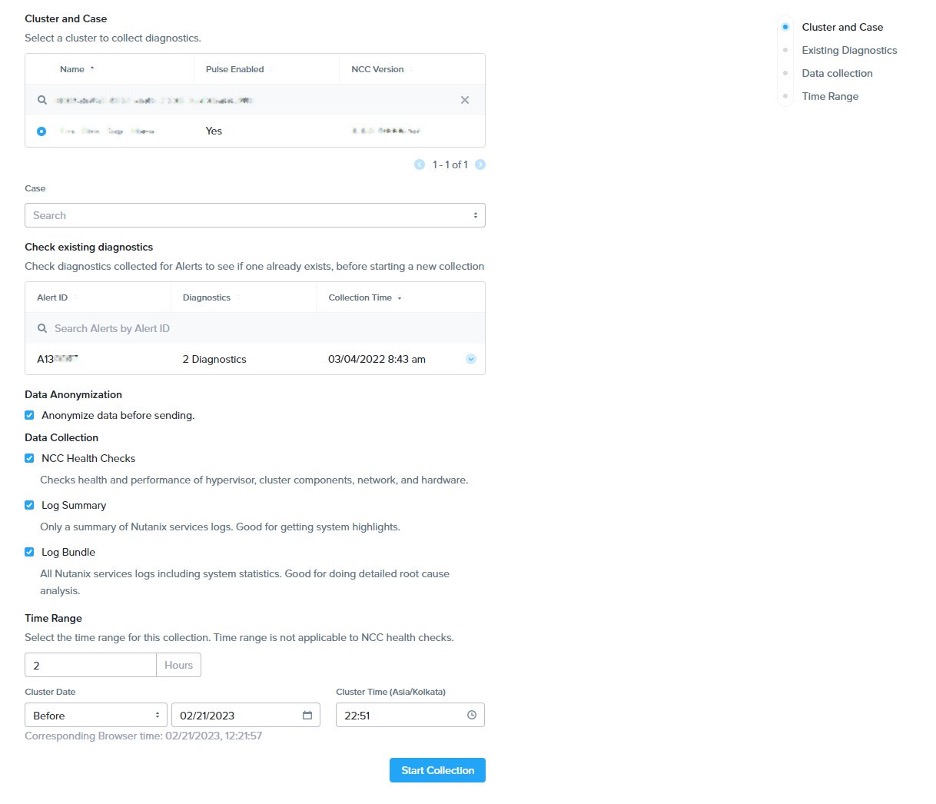This image showcases a section of a company’s website dedicated to diagnostics and data analysis. On the top left corner, the webpage begins with options related to “Cluster” and “Case” for diagnostics collection. The following sections are organized into categories, showcasing different functionalities:

1. **Cluster Selection and Diagnostics Collection**:
   - **Top Left Corner**: “Cluster” and “Case” selections for initiating diagnostics collection.
   - **Below Cluster Selection**: Various categories including:
     - **Name**: A field for the name category.
     - **Pulse Enabled**: A field for pulse status.
     - **NCC Version**: Version information.

2. **Search and Input Fields**:
   - **Rectangle Box**: Immediately below the categories, there is a long rectangular search box featuring a magnifying glass icon on the left and a close (X) button on the right. The text inside this box is blurred.
   - **Blue Circle**: Below the search box, there is a blue circle with a white dot at its center, containing blurred text, but with a distinguishable “Yes” in the middle.

3. **Case Section**:
   - **Search Box**: Below the blue circle section, the “Case” section starts, which includes a search box with an up or down arrow for navigation.
   - **Check Existing Diagnostics**: An option followed by fields for alert ID, diagnostics, and collection time.
   - **Search Alerts by ID**: Instructions for searching alerts using ID.

4. **Data and Anomalization Section**:
   - **Data Analysis**: This section follows with options for analyzing data before sending.
   - **Data Collection Checkboxes**: All options under this section (like “Analyze data before sending”) are checked.
   - **Time Range and Input Fields**: It includes a time range option with associated information and four input boxes for data entry.

Overall, the webpage provides a structured interface for collecting, searching, and analyzing diagnostic data, detailed with multiple categories and search functionalities.